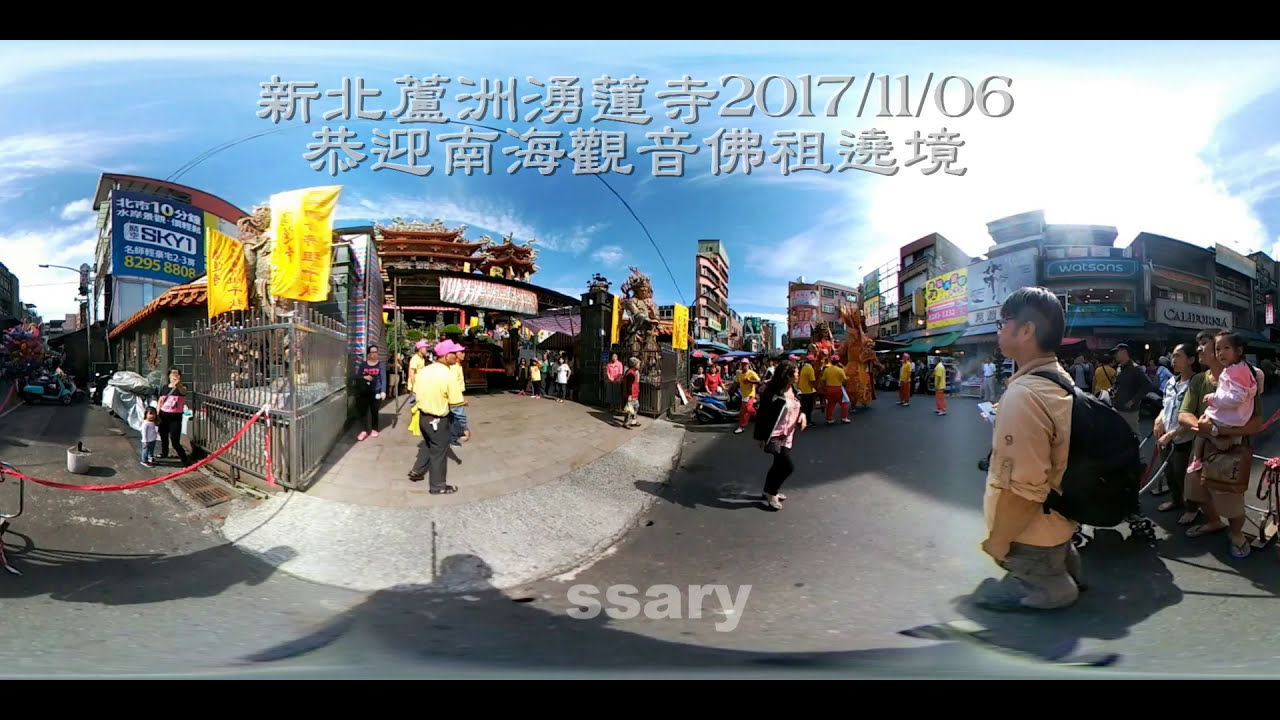This horizontal rectangular image, framed with thin black borders at the top and bottom, captures a bustling scene in what appears to be an Asian city on a bright, clear day. At the top of the image, there are Chinese characters and the date "2017-11-06." Beneath this text, the image presents a lively street market with colorful signs dominating the smaller buildings. The streets are crowded with people, some carrying backpacks, purses, and wearing various types of headgear, including ball caps. Prominently to the right, a person with a backpack leans on a fence, while other figures, potentially workers in yellow shirts, mingle and move within the bustling scene. In the background, taller buildings loom over the market, illustrating the mix of traditional and modern architecture. The image exhibits a convex distortion, possibly from an unusual lens, creating circular patterns throughout. The sky above is a bright blue with a few clouds, reinforcing the sense of a vibrant, thriving marketplace.